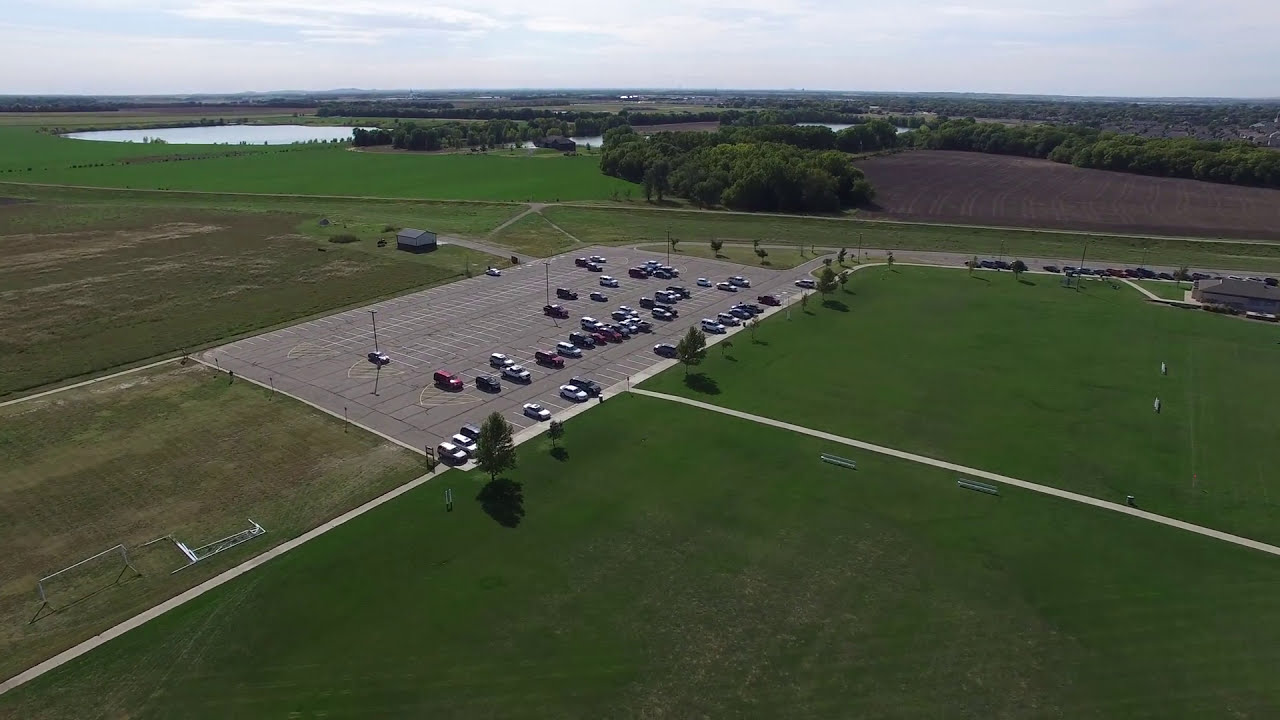This aerial photograph captures a large, triangular-shaped parking lot positioned slightly to the left but central within the image. The lot, which appears to be approximately a third full, hosts a variety of cars in red, white, black, and other colors. Surrounding the parking area are well-manicured green lawns, with a notable lack of trees except for some distant ones. 

In the distance on the left side of the image, a small lake framed by green trees can be seen, adding a touch of natural beauty to the scene. Adjacent to the parking lot, several roads converge, intersecting the green areas perpendicularly. Despite their prominence, these roads appear devoid of moving vehicles. 

Further beyond the parking lot, there are different fields and dirt areas, suggesting agricultural use, with boundaries clearly marking private properties. A solitary house with a road leading to it and a building, possibly a business with its own parked cars, also feature in the composition.

Up in the sky, a mostly cloudy horizon with shades of white and gray adds an overcast ambiance to this daytime shot. There is a pathway intersecting the green expanses, hinting at possible recreational use, while a barn-like structure nestles in the far background, blending with the landscape's rural character.